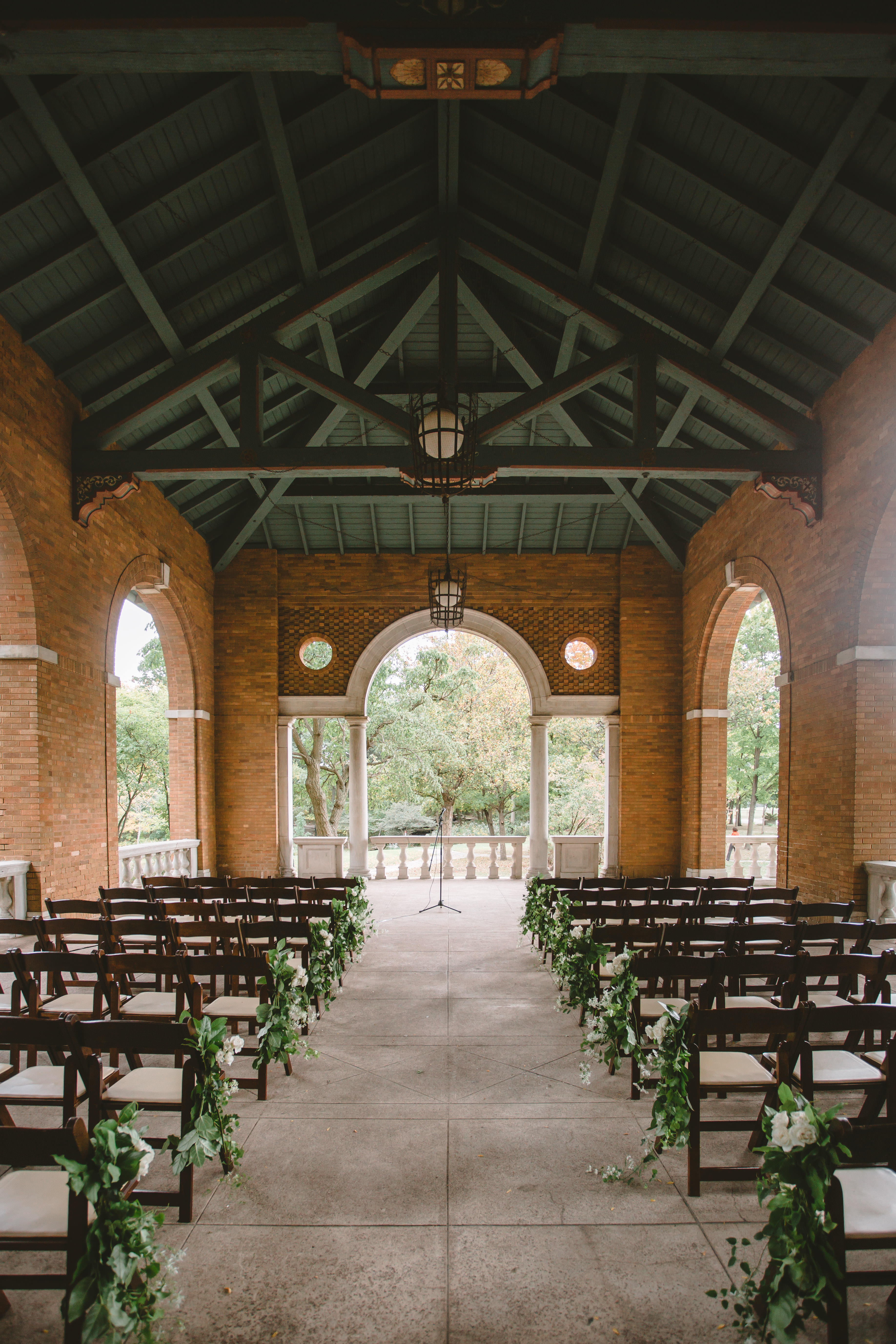The image depicts a beautiful, open-air wedding venue that resembles a chapel or amphitheater with a distinctive blend of rustic and elegant elements. The space features high, green-painted rafters and a wooden green roof adorned with rustic lighting. The walls are constructed of amber bricks with large, arch-shaped openings, giving it a semi-enclosed feel. The floor appears to be made of textured stone or cement. The venue is set up with several rows of dark wooden folding chairs, each with light-colored or white cushions. Floral decorations composed of white and green arrangements adorn the aisle-end chairs. At the front of the venue, white columns and a white railing complement the minimalist but sophisticated decor. A microphone stand is positioned at the end of the aisle, indicating the designated spot for the officiant. The overall ambiance is serene and picturesque, ideal for an intimate wedding ceremony.